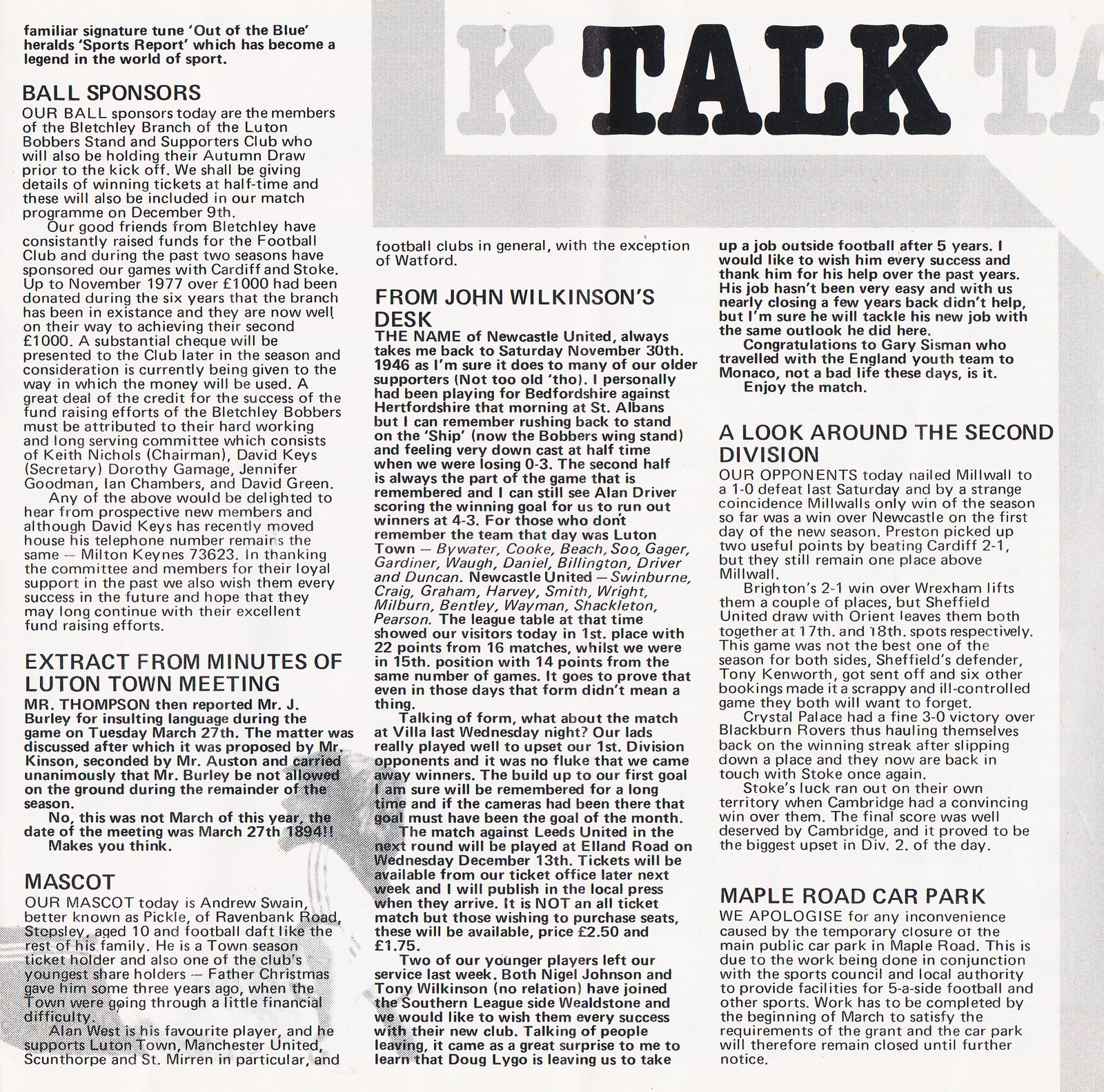The image is a cut-out from a newspaper or magazine page. At the top right, it prominently features the text "Ktalk TA." The article includes several sections, each with its own heading. On the top left, the first section is titled "Bold Sponsors," detailing the current support from the Beech Lead Branch of the Luton Bobbers Stand and Supporters Club, which is actively engaging in fundraising for the football club. Below this, one section is "Extract from Minutes of Luton Town Meeting," and underneath it, there is another section titled "Mascot," presumably discussing details about the mascot for the day's event. In the middle column, there's a section titled "From John Wilkinson's Desk," offering insights or updates from a notable individual. On the right side, there's a section called "A Look Around the Second Division and Maple Road Car Park," which provides information on the second division and local facilities. The background of the image is primarily white or light gray. In the bottom left corner, a silhouette of a person is faintly visible, though it blends into the writing, making it difficult to distinguish. The article further mentions a familiar signature tune, "Out of the Blue," linked to Harold's sports report, which is famed in the sporting world.